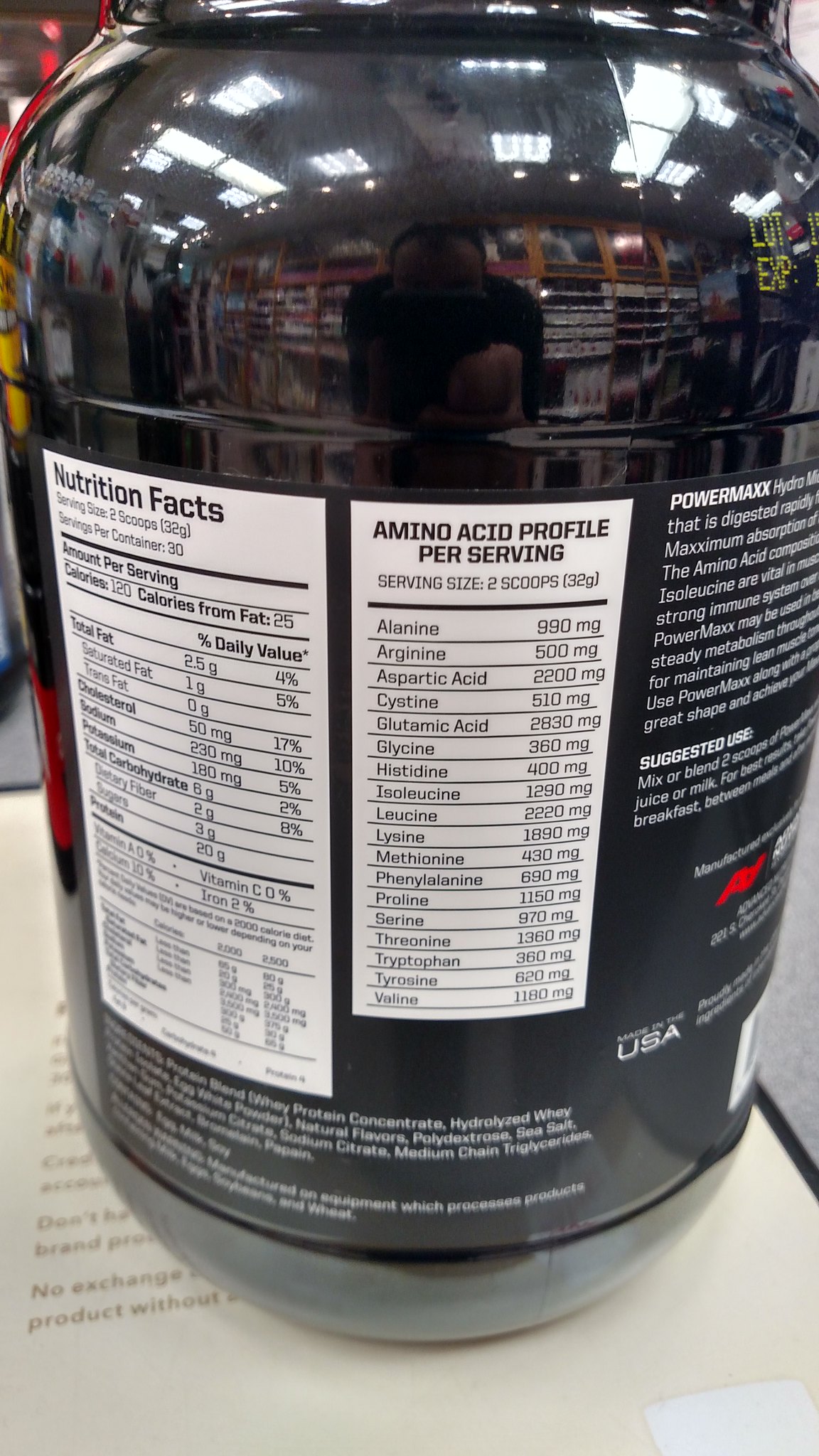The image depicts the backside of a black plastic bottle, likely containing protein powder branded as PowerMax. Prominently featured on the bottle is a large white rectangular area displaying nutritional facts. Adjacent to this, another white rectangular section details the amino acid profile per serving. To the right, there is additional informational text discussing performance, followed by further text at the bottle’s bottom, presumably listing the ingredients. At the top of the bottle, an image shows a person behind a shopping cart with the aisles of a grocery store reflected in the background. The bottle is sitting on a piece of paper, and the scene appears to be located on a counter inside a wholesale club, potentially a Sam's or Costco, with shelving visible behind the reflected individual. The product is noted to be made or distributed in the USA.